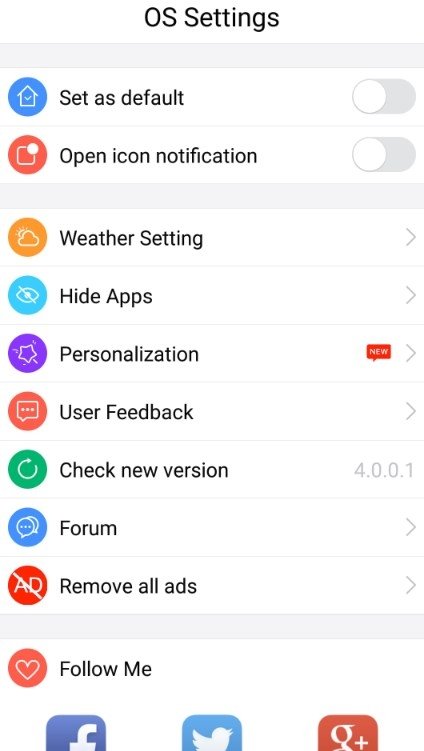The image features a white background with a series of organized sections:

1. **OS Settings**: Positioned at the top.
2. **Default Home Setting**:
   - A small blue box.
   - Below it, there’s a blue circle with a house icon labeled "Set as Default."
   - Accompanied by a toggle switch.
3. **Notification Settings**:
   - A red circle with a square inside it, containing a small white dot labeled "Open Icon Notification."
   - Followed by another toggle switch.
4. **Additional Settings**:
   - A white box containing:
     - "Weather Settings"
     - "Hide App"
     - "Personalization" with a red box labeled "NEW" on the right.
     - "User Feedback"
     - "Check out new version 4.0.0.1"
     - "Forum"
     - "Remove all ads"
   - Each category ends with a right-arrow icon.
5. **Social Media Section**:
   - Another white box with a red circle and a heart icon labeled "Follow Me."
   - Followed by icons for Facebook, Twitter, and Google+.